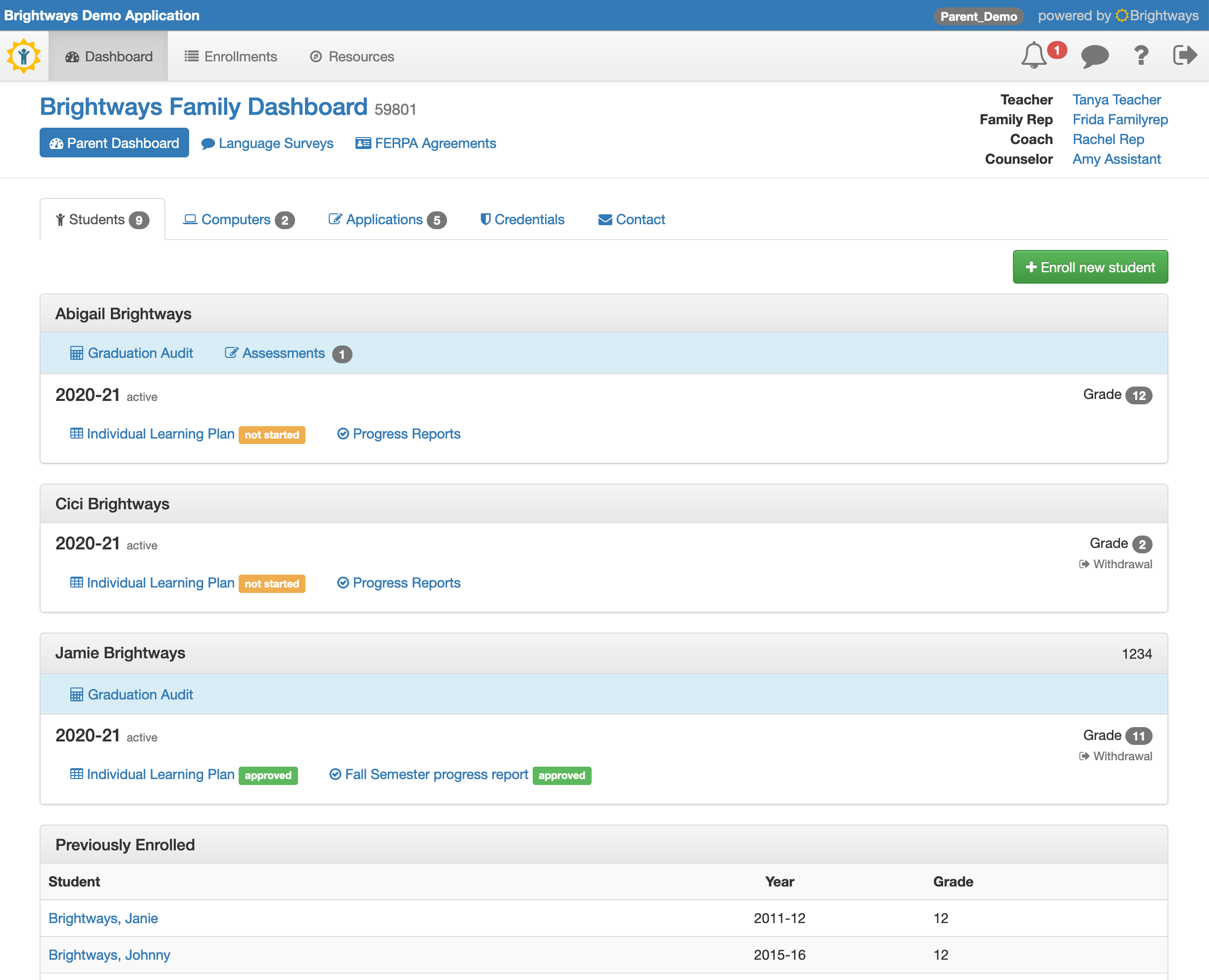**Bright Ways Demo Application Interface**

The image depicts a comprehensive interface for the Bright Ways Demo Application, which appears to be a prototype for a teacher's grading and reporting site. The layout is designed to provide educators and associated staff with a detailed overview of student information, progress, and related resources.

**Header:**
- A prominent blue bar at the top features the application name "Bright Ways Demo Application" in white, positioned on the upper left.
- Within the blue bar, a greenish oval with white text reads "Parent Demo".
- To the right, the phrase "Powered By" accompanies an orange circle and the words "Bright Ways" in gray letters.
- On the upper right, a yellow circular icon with short spikes and a person silhouette is visible.

**Navigation and Icons:**
- Below the blue bar, multiple navigation tabs are highlighted, including "Dashboard", "Enrollments", and "Resources".
- On the topmost bar:
  - A bell icon with a number '1', signaling notifications.
  - A speech bubble icon in gray containing a question mark, followed by an arrow symbol pointing right with a bracket to its left.
  - The text "Bright Ways Family" in blue, followed by "Family Dashboard" and "59801" in black letters to the right.

**Parent Dashboard Section:**
- Highlighted options include "Parent Dashboard" with a dashboard icon, "Language Surveys" with a speech bubble, and "FERPA" represented in a blue and white rectangular icon.
- To the far right, roles like "Teacher", "Family Rep", "Coach", and "Counselor" are listed in black, showcasing demo names like Tanya Teacher, Frida Family Rep, Rachel Rep, and Amy Assistant in blue.

**Student Information:**
- A gray tab titled "Students" with a number '9' in a gray circle is open, listing student names like Abigail Brightway, Cece Brightway, and Jamie Brightway in black.
- Tabs for "Computers" (blue computer icon, '2'), "Applications" (blue square with paintbrush icon, '5'), "Credentials" (shield icon), and "Contact" (envelope icon) are also present.

**Student Enrollment and Reports:**
- A green box with a plus mark and white text labeled "Enroll New Student" is positioned towards the bottom right.
- Below, gray bars list student progress details such as year (2020-21), status (active), and grades (12, 2, 1, 11) with a focus on key assessments:
  - Graduation Audit (blue bar at top and bottom of some entries).
  - Various individual learning plans, progress reports, and statuses like "Not Started" in orange or "Approved" in green.

**Historical Data:**
- Past enrollment data, including "Previously Enrolled" and students like Jamie and Johnny Brightway, with years (2011-12, 2015-16) and grades, are also indicated.

This detailed layout serves as a valuable tool for educators to monitor and manage student progress effectively, reflecting the functionality and design considerations tailored for educational reporting and administrative tasks.